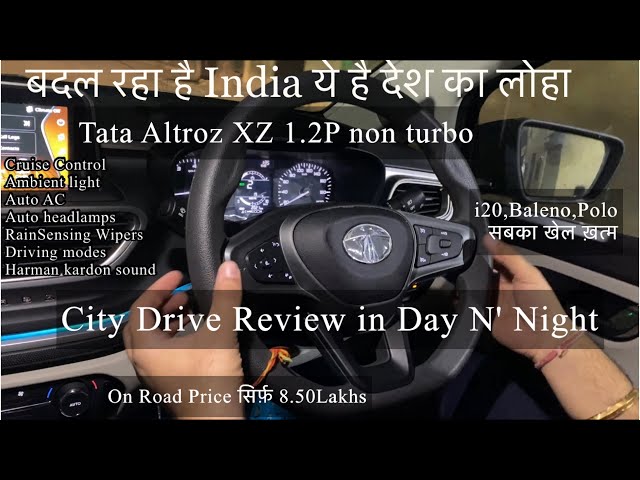The image showcases the interior of a Tata Altroz XZ 1.2P non-turbo, a right-hand drive car. The main focus is the black steering wheel, which bears the Tata logo and is held by a person with visible hands adorned with some jewelry. Behind the steering wheel, the black dashboard is prominent, featuring a speedometer and clear white text. The text includes terms such as "City drive review in day and night," "On-road price: 8.50 LAKHS," and various car features like "cruise control, ambient light, auto AC, auto headlamps, rain sensing wipers, driving modes, and Harman Kardon sound." Surrounding these elements, there's a black rectangular border with additional white text in a foreign language, likely Indian, mentioning "India" and "Tata Altroz XZ 1.2P non-turbo." The image provides a detailed look at the car's interior features and specifications, highlighting both the design and textual information about the vehicle.